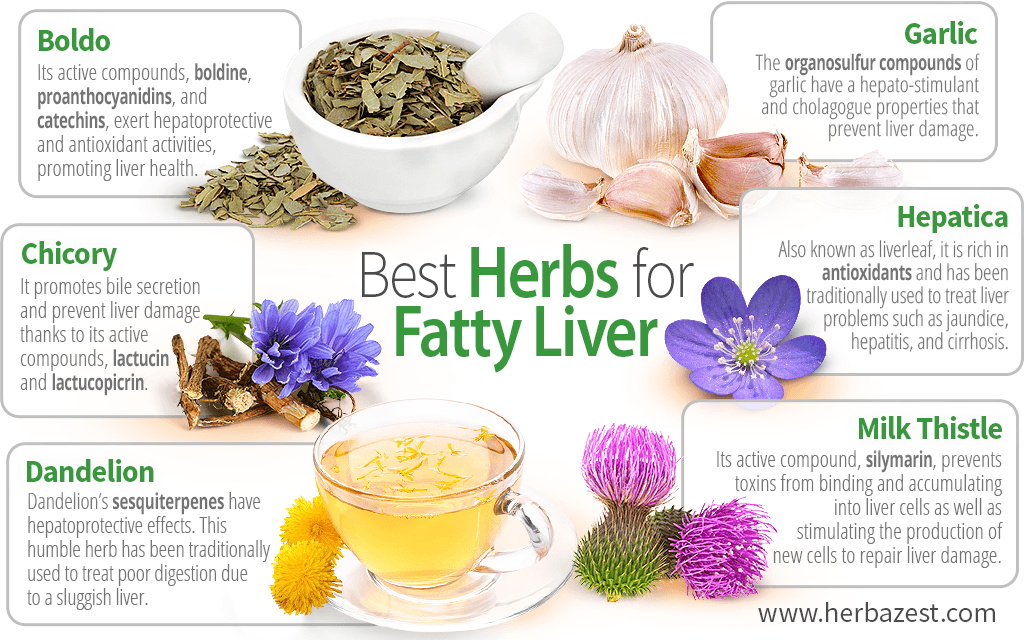The infographic, set against a white background, is titled "Best Herbs for Fatty Liver" prominently in the center. Surrounding the title are detailed images of various beneficial herbs, each accompanied by text blocks providing brief descriptions of their liver-supporting properties. 

On the left side, the top image features a white bowl filled with dried boldo, commonly used for its detoxifying effects. Below it, the next block depicts chicory, showcasing its root and blue flower, known for aiding digestion and liver function. The third block on the left shows a clear glass cup on a glass saucer filled with yellow dandelion tea, an herb praised for its cleansing properties.

On the right side, the top image displays a bulb of garlic, celebrated for its anti-inflammatory and liver-protective qualities. Below garlic is hepatica, illustrated with its distinct purple flower, used traditionally for liver health. The bottom right block features milk thistle, with green buds and pink flowers, well-regarded for its active compound silymarin that supports liver regeneration.

Each herb is depicted in a form that highlights its unique characteristics, such as dried leaves, flowers, or beverages, making the infographic not only informative but visually engaging.